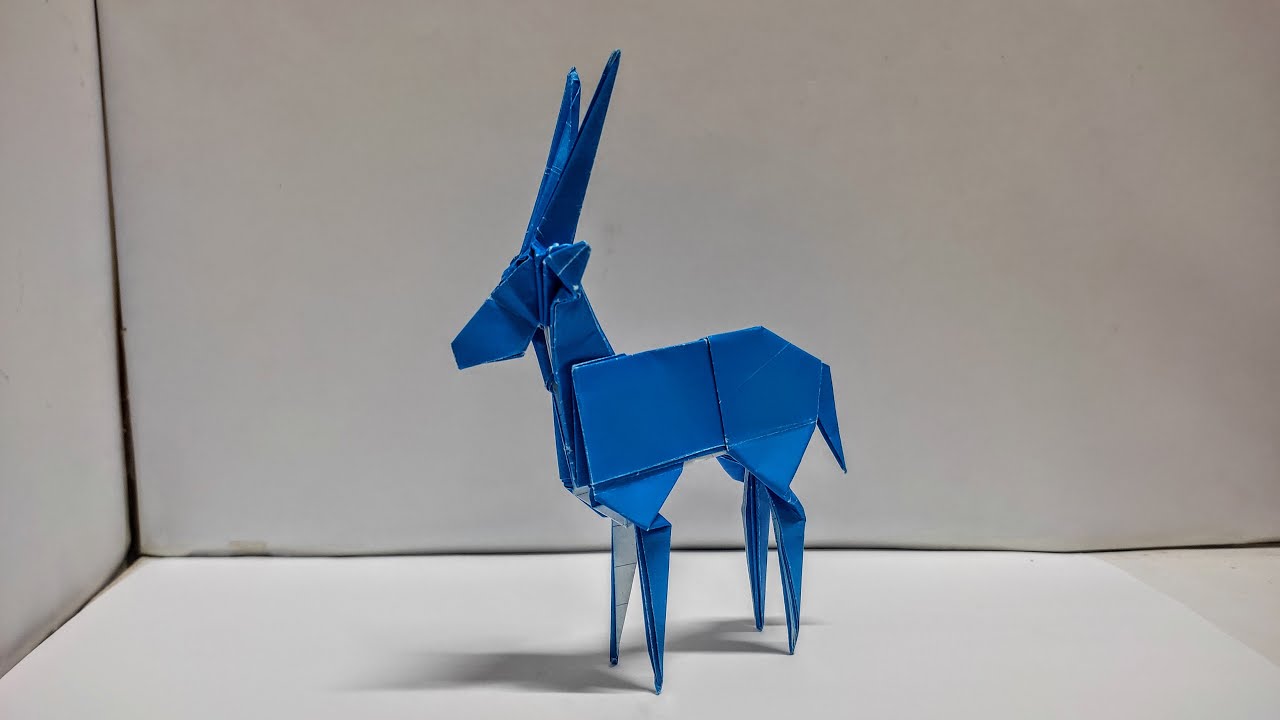The image showcases a detailed photograph of a modern art piece—a blue origami-style sculpture resembling an antelope or a deer, characterized by its distinctive large ears and pointed horns. The artwork is meticulously crafted, seemingly from plastic or metal sheets, giving it a sleek, contemporary look. It stands prominently on four legs on a stark white surface, with a white background that appears almost like the inside of a box, enhancing the minimalist aesthetic. Notably, one of the legs features a silver trim, adding a subtle contrast to the predominantly blue structure. Shadows and lines, including a notable Y-shaped shadow, contribute to the depth and intrigue of the image, while the overall clean and monochromatic setting emphasizes the centrality and elegance of the antelope-like figure.